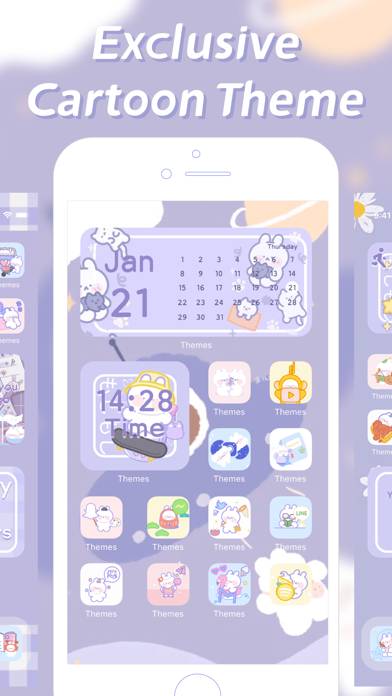The image captures a vibrant screenshot showcasing various cartoon-themed backgrounds for cell phones. The backdrop of the image is a serene light blue sky adorned with fluffy white clouds that cluster near the top, giving it an airy feel. On the upper right side, a radiant yellow sun peeks into the frame, casting a warm glow.

Dominating the upper section of the screenshot, bold white letters spell out "Exclusive Cartoon Theme," highlighting the uniqueness of the offerings. The centerpiece of the display is a prominent background featuring a delightful array of cartoon animals each associated with different icons. These themes are represented within individual squares, each meticulously labeled as "themes."

In the middle of these thematic squares, the time "14:28" is conspicuously displayed inside a larger square, with the word "time" elegantly positioned underneath it. This larger square stands out as the focal point amidst the smaller ones, emphasizing the central theme. Notably, there is a conspicuous absence of additional text, suggesting a deliberate choice possibly to avoid copyright issues.

Overall, this screenshot is a cheerful and engaging representation of cartoon-themed cell phone backgrounds, blending playful imagery with functional design elements.